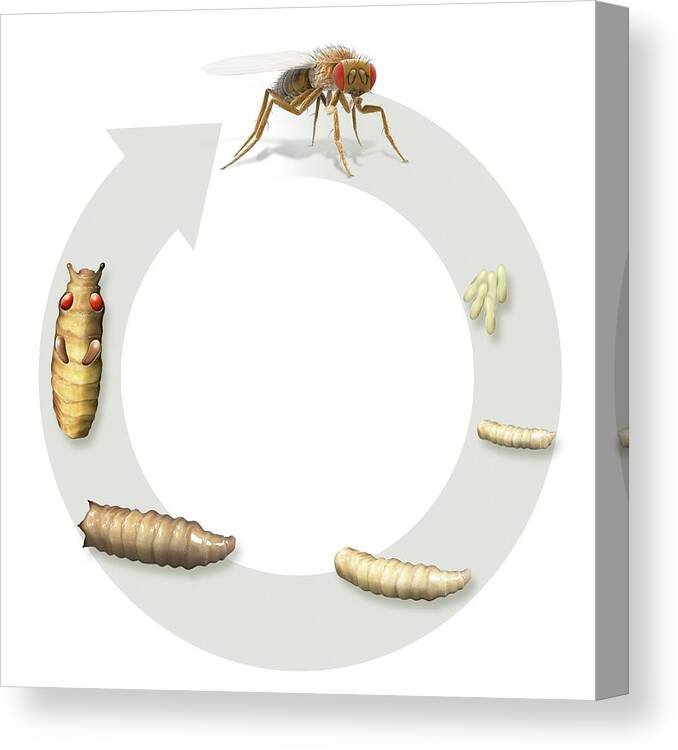This is a detailed digital illustration, designed to resemble a canvas hanging on a wall, depicting the life cycle of an insect. The canvas is viewed slightly from the side, showing its depth against a white background. At the centerpiece of this square canvas is a large, light gray circular arrow that frames the cycle.

Starting at the top of the canvas, the illustration begins with a cartoon-like adult fly, distinguished by its red eyes and dark wings. Moving clockwise, the cycle transitions through five distinct stages: eggs, progressively larger larvae, and a sequence of cocoons, each stage growing and developing more than the last. The final cocoon stage shows the emergence of an adult fly with hints of antennae and legs visible, completing the cycle.

The artwork uses a palette that includes light gray, white, brown, red, and black, emphasizing the stages without text labels. The meticulous shadowing enhances the depth, giving the illusion that this digital piece is an unframed painting on canvas.